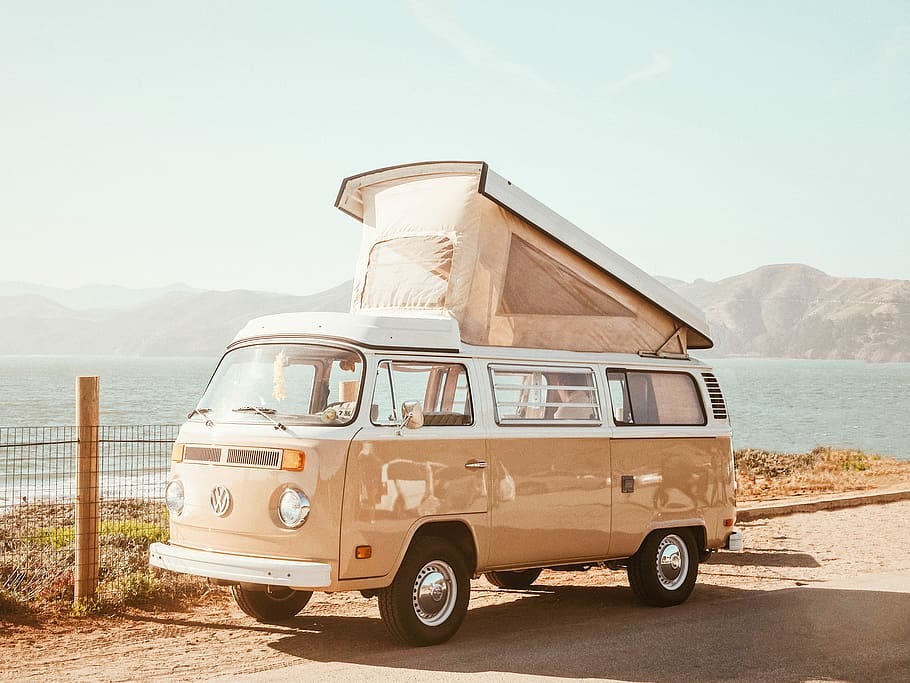The image depicts a classic VW minivan with a pop-up camper, situated by the ocean, with a faint dusky blue sky in the background. The minivan showcases the iconic VW logo at the center front and is characterized by its almost flat front. The bottom portion of the vehicle is a shiny light tan, while the top is white. The pop-up camper tent on top of the minivan is beige and triangular in shape, featuring screened windows at the front and side. A man is visible inside the tent. Between the vehicle and the ocean, there is a metal fence. The ground appears to be made of dirt, and mountains can be seen faintly in the background.